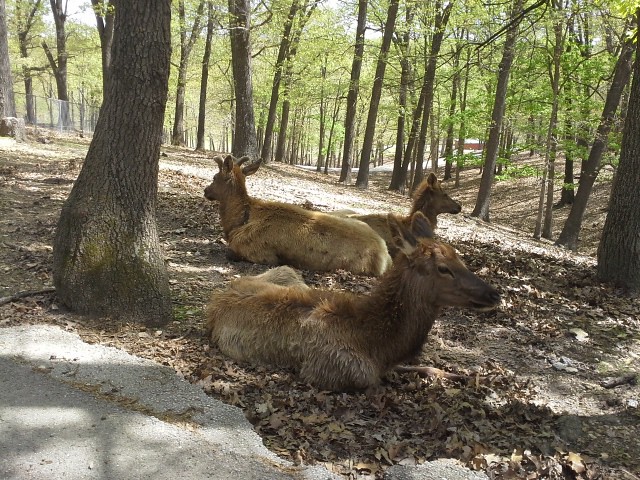In the foreground of the image, three mammals, resembling deer or antelopes with characteristics of thin muzzles and teardrop-shaped eyes, are lying on a ground covered with brown, crispy leaves and light gray gravel. Their fur is predominantly brown, with two of the animals facing to the right and one, lighter coated, facing to the left, showcasing its short, curving horns. Encircling their resting area are sparse deciduous trees with slender trunks, some still clinging to green leaves amidst the predominantly brown foliage, indicating a transitional season. In the background to the left, a tall chain-link fence is visible, hinting the enclosure might be within a kept or managed environment. A patchy combination of dappled sunlight and shade scatters across the scene, and small glimpses of a light blue sky can be seen through the canopy of thin branches and leaves.